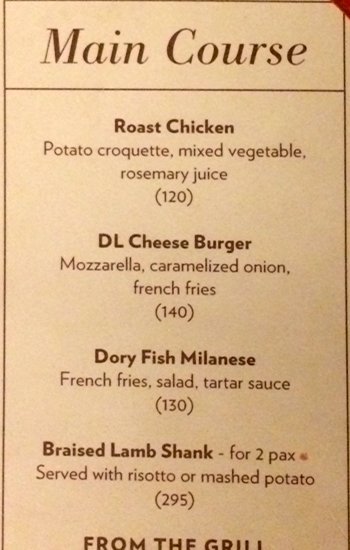The image depicts a section of a menu presented on tannish-colored paper. In the upper right-hand corner, there is a red triangle, suggesting the paper is held in a red holder. Across the top, "MAIN COURSE" is prominently displayed in large letters, underlined the full width of the paper. Below this heading, the menu items are listed as follows:

- **Roast Chicken**: Described with "potato croquette, mixed vegetable, rosemary juice," followed by "(120)" indicating its order number.
- **DL Cheeseburger** (in darker print): Includes "mozzarella, caramelized onion, french fries," with "(140)" as its order number.
- **Dory Fish Milanese**: Accompanied by "french fries, salad, tartar sauce," and "(130)" next to it.
- **Braised Lamb Shank**: Marked with a dash, indicating "42 PAX," and detailed with "served with risotto or mashed potato," followed by "(295)".

At the bottom of the image, "FROM THE GRILL" is displayed in large capital letters, although some of the letters are partially cut off due to the image's cropping. The text across the menu appears to be in red print.